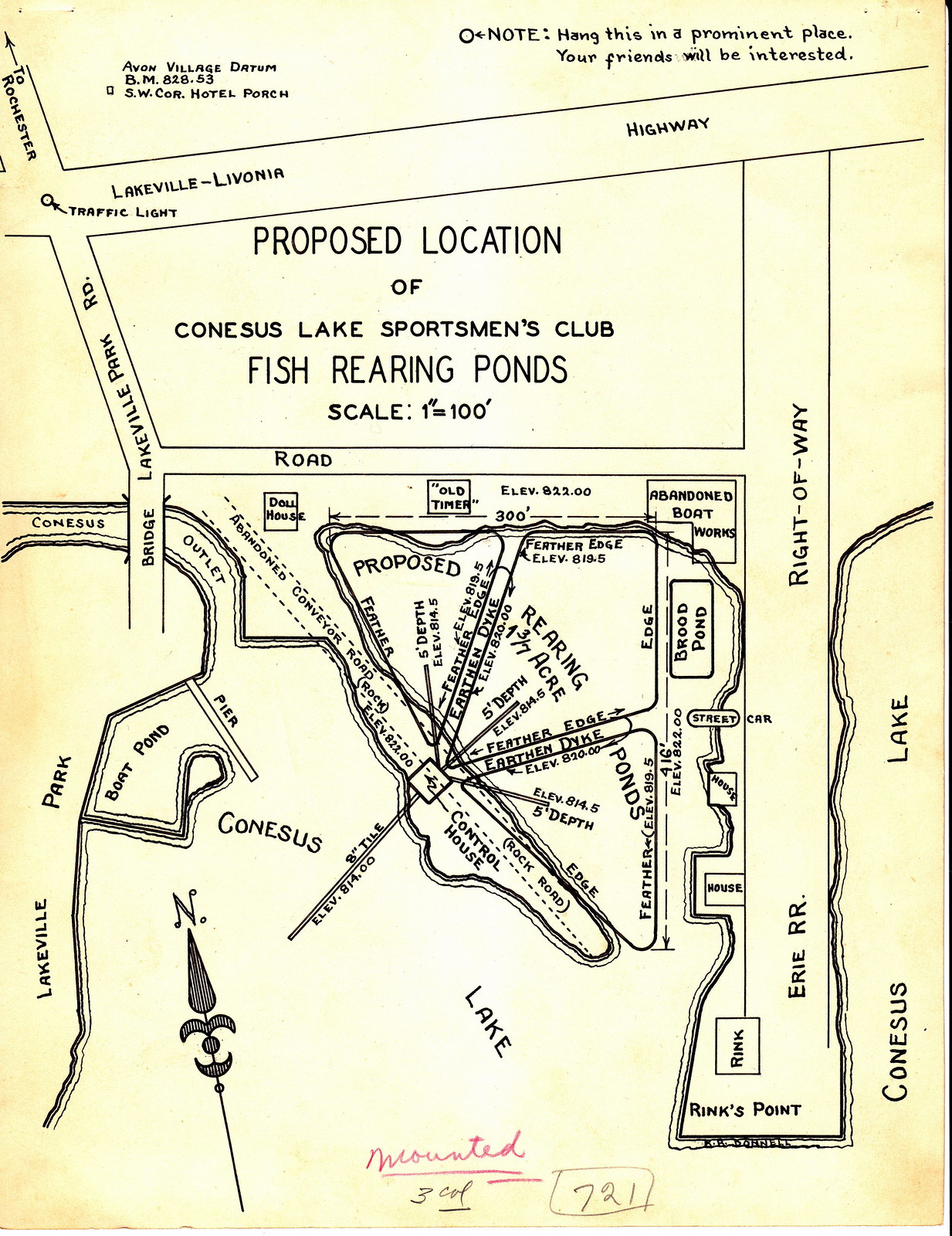This vertically oriented graphic, titled "Proposed Location of Conesus Lake Sportsman's Club Fish Rearing Ponds," serves as a detailed map with a scale of 1 inch equaling 100 feet. At the top of the map, there's the Erie Railroad right-of-way crossing horizontally, while a vertical road labeled 'Plain Road' runs down the right-hand side. The intersection of Lakeville-Lavonia Road Highway and Lakeville Park Road is marked by a traffic light, with Lakeville Park and a boat pond nearby. Conesus Outlet is also depicted on the map.

The proposed fish rearing ponds are centrally located, surrounded by earthen dikes and a control house. The label notes that a portion of Conesus Lake may be drained for these ponds, which are detailed with various dimensions. Towards the bottom center of the map, an arrow points due north. Handwritten notes include "Mounted and 3 Cole 721."